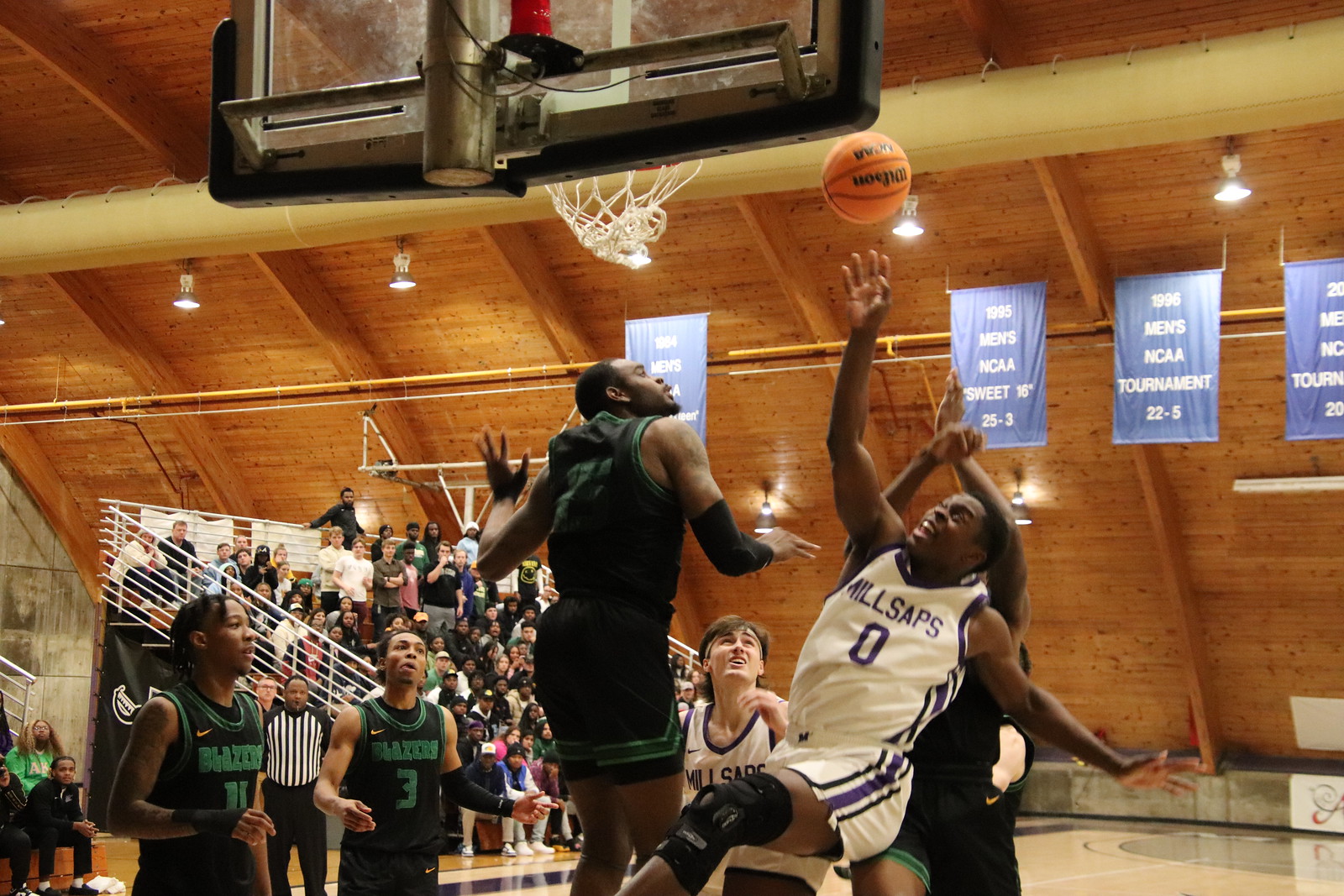This is a detailed action shot photograph taken during a basketball game between two teams, identified as the Blazers in black and green uniforms and the Millsaps in white and purple uniforms. The image captures an intense moment near the hoop from a viewpoint behind the backboard. The main focus is on three players in white and black uniforms at the forefront. One player in a white uniform, who is wearing a knee brace, appears to be falling while tossing the basketball towards the hoop; the ball is about six inches above his hand, suggesting he just released it. Two players in dark uniforms surround him—one directly in front of him and another behind, both also engaging in the play.

The ball seems to be in middle action, possibly heading towards the basket, indicated by the net fluttering upwards. The scene is set in an indoor gym, evidenced by the visible wooden rafters and accompanying banners proclaiming past NCAA tournament achievements from 1995 and 1996. The background features small bleachers filled with spectators, reinforcing the atmosphere of a spirited high school or college basketball game.